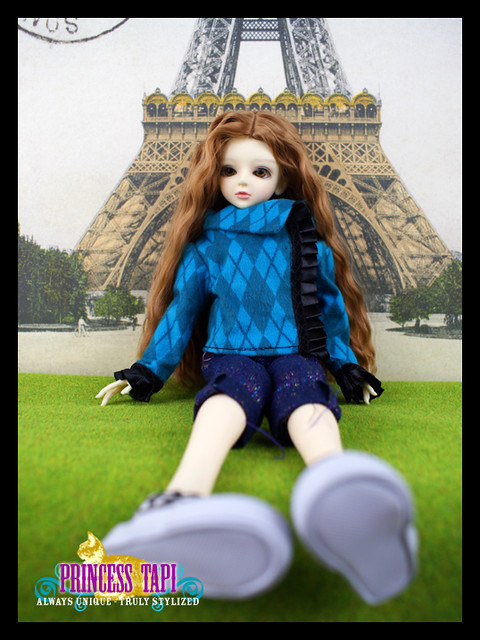This photograph features a light-skinned doll positioned in front of an image of the Eiffel Tower, creating an embodiment of a postcard scene. The background appears to depict either a real or illustrated Eiffel Tower, enhancing the postcard-like aesthetic with a partial postmark in the upper left corner and the phrase "Princess Tuppy, always unique, truly stylized," inscribed in the lower-left corner. The doll is seated on a green grass-like surface, possibly astroturf or felt, with her legs stretched out towards the camera. She wears a dark blue and medium blue diamond-patterned top with distinctive lacing details and matching denim-like shorts that reach her knees. Her sneakers, with gray soles, appear prominently in the foreground, emphasizing their proximity to the camera lens. The doll has long, waist-length, curly auburn hair, and she gazes slightly to the left. Her eyes, a deep brown, are fixed in an off-camera glance, rounding out the scene's whimsical composition.